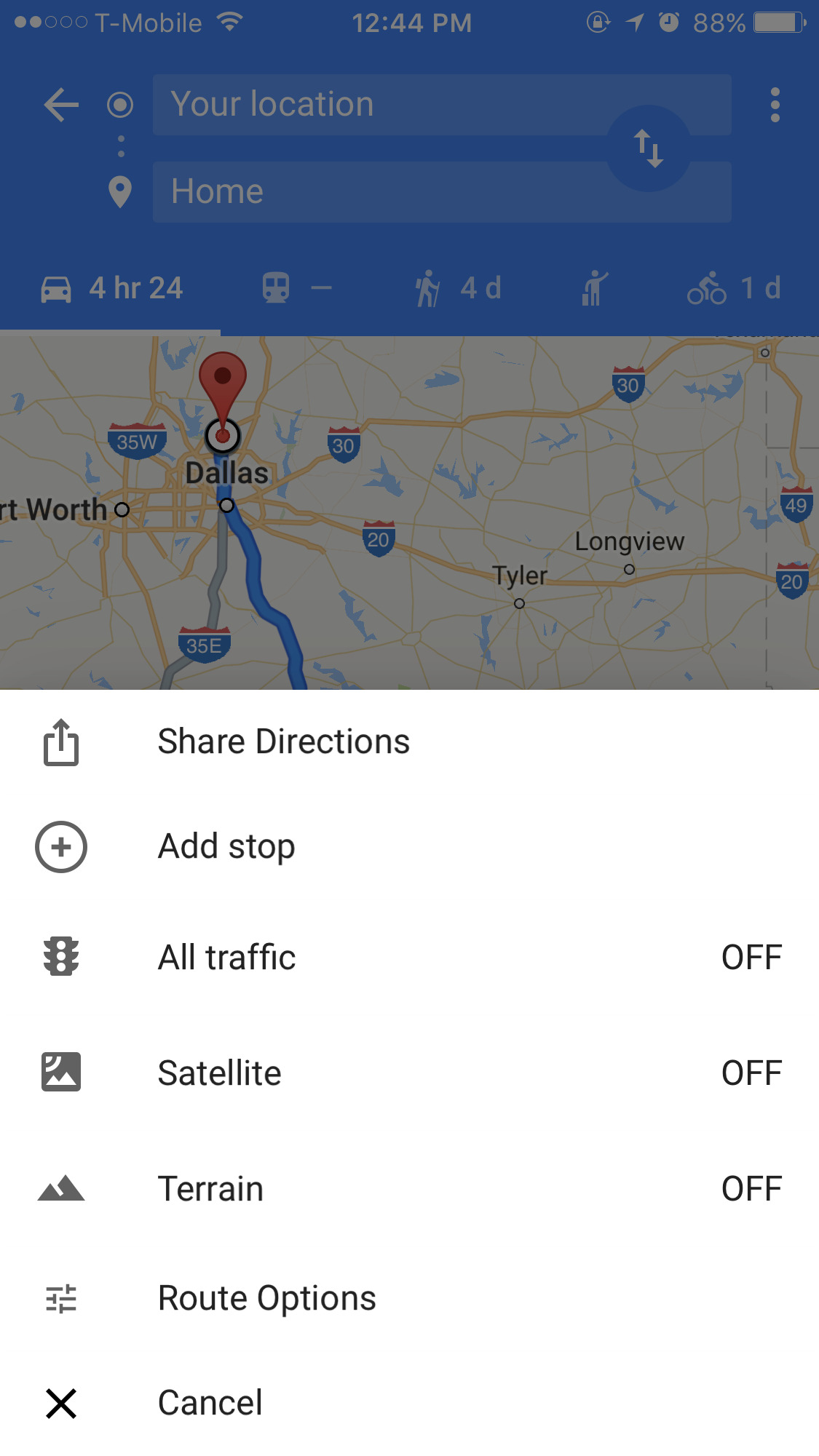This is a detailed screenshot of a partial map of Dallas, Texas. The city is marked with a prominent red bubble containing a black dot, with the name "Dallas" clearly labeled in black text. The map extends to include portions of Fort Worth, which is also labeled. Major highways are indicated, with Route 35W situated to the left (west) of Dallas, Route 35E positioned to the south, and Routes 20 and 30 shown to the right (east) of Dallas. Additionally, the towns of Longview and Tyler, Texas are visible, along with Routes 49 and 20.

Below the map, a menu displays various navigation and map options: 
- "Shared Directions" is represented by a square with an up arrow.
- "Add Stop" features a circle with a plus sign.
- "All Traffic," marked with a traffic light icon, is shown as off.
- "Satellite," though the specific icon is unclear, is also marked as off.
- "Terrain," represented by a mountain icon, is off as well.
- "Route Options," depicted by arrows pointing left and right.
- "Cancel," identified by an X icon.

Each category in the menu has a corresponding icon to the left of it, enhancing the user interface for easier customization of the map’s display and route planning.